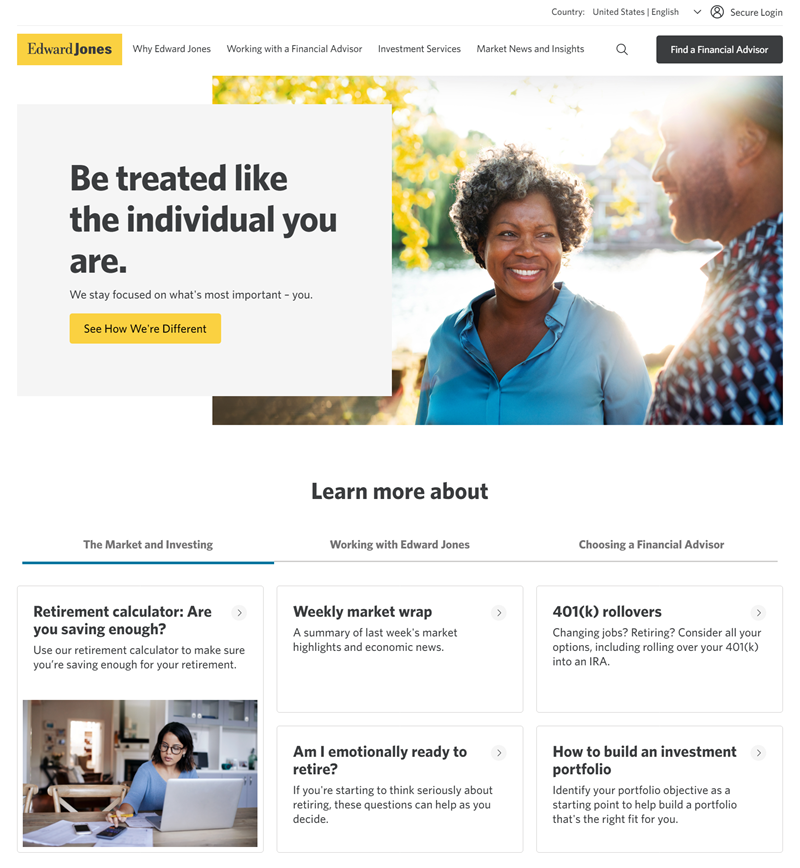The image depicts a diverse group of individuals engaging with various financial services offered by Edward Jones. In the foreground, a man and a woman stand next to each other; the man wears a black and blue checkered shirt, while the woman is dressed in a blue shirt. Additionally, another woman in a blue shirt is focused on her silver-colored laptop as she sits at a table, presumably reviewing her investments or retirement plans.

The backdrop emphasizes Edward Jones' commitment to personalized financial advising, with phrases like "Be treated like the individual you are" and "See how we're different." The services highlighted include investment portfolios, 401k rollovers, retirement calculators, and emotional readiness for retirement. The scene underscores the various tools and resources available, such as secure login and market news, aimed at helping clients in the United States make informed financial decisions. The overall vibe suggests a supportive and personalized approach to financial planning.